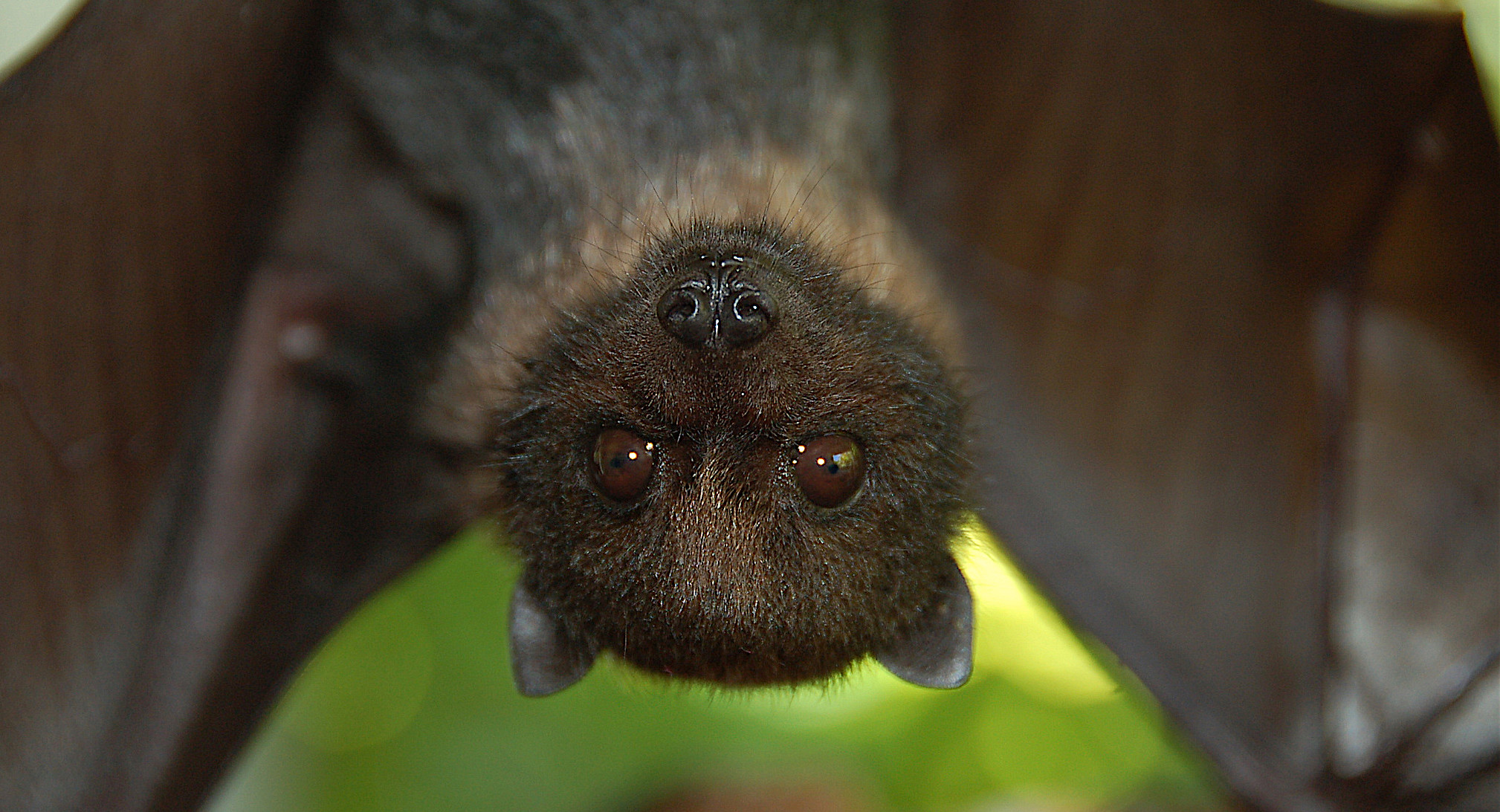This close-up photograph captures a detailed view of a bat hanging upside down, showing it from the chest up. The bat sports a dark brown, fuzzy face with large, dark eyes resembling a coffee hue and small black irises. Its black, wet nose and dark, pointed ears can be distinctly seen, adding to the bat's endearing appearance. The bat's chest fur is a lighter brown interspersed with some white hairs, giving it a textured look. Its wings, which spread out behind it in an upside-down V shape, are dark brown and reveal the underlying bone structure. The background is slightly blurry with a green hue, suggesting the bat is in its natural environment. The backdrop is largely made up of the bat's wings, framing the image on both sides, with a bit of the green background visible behind its head.